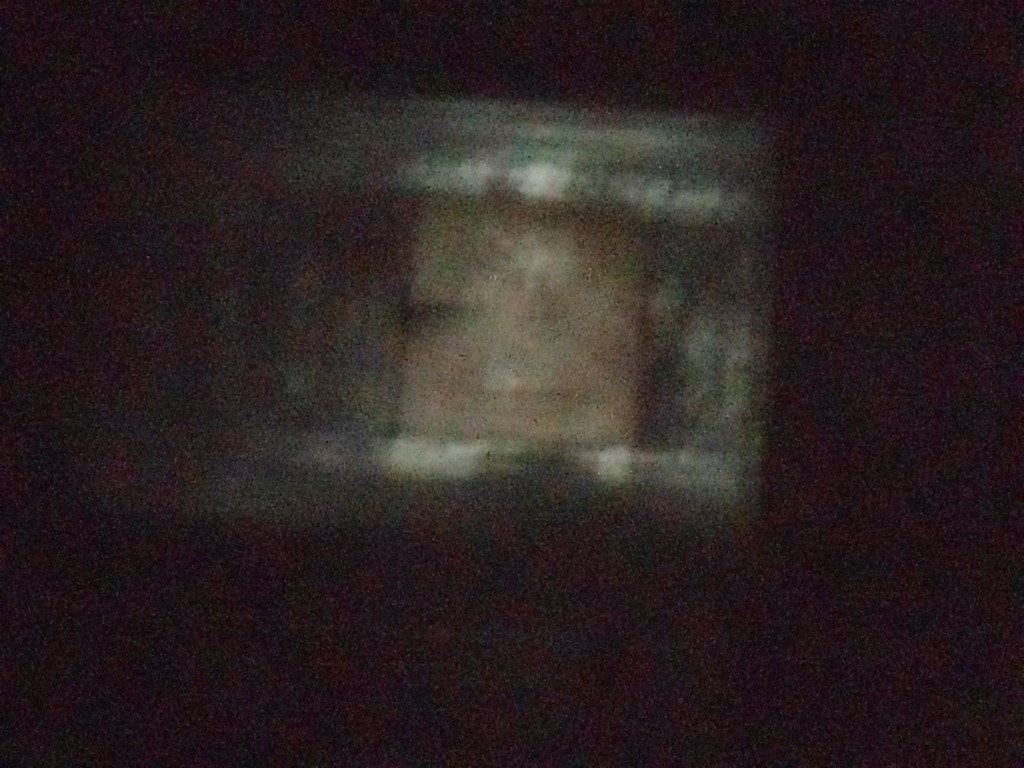The image portrays a dark and grainy scene, dominated by an unidentifiable central object. This object, which appears to be a gray rectangle with potentially ridged edges, contrasts starkly against the near-black background. The rectangle houses a smaller, peach or beige-colored interior box. Scattered across the dark backdrop are small, blotchy patches of lighter yellow, hinting at faint reflections of light rather than the application of a filter. The overall composition is marked by obscurity and minimal illumination, creating an enigmatic and somewhat abstract visual experience.